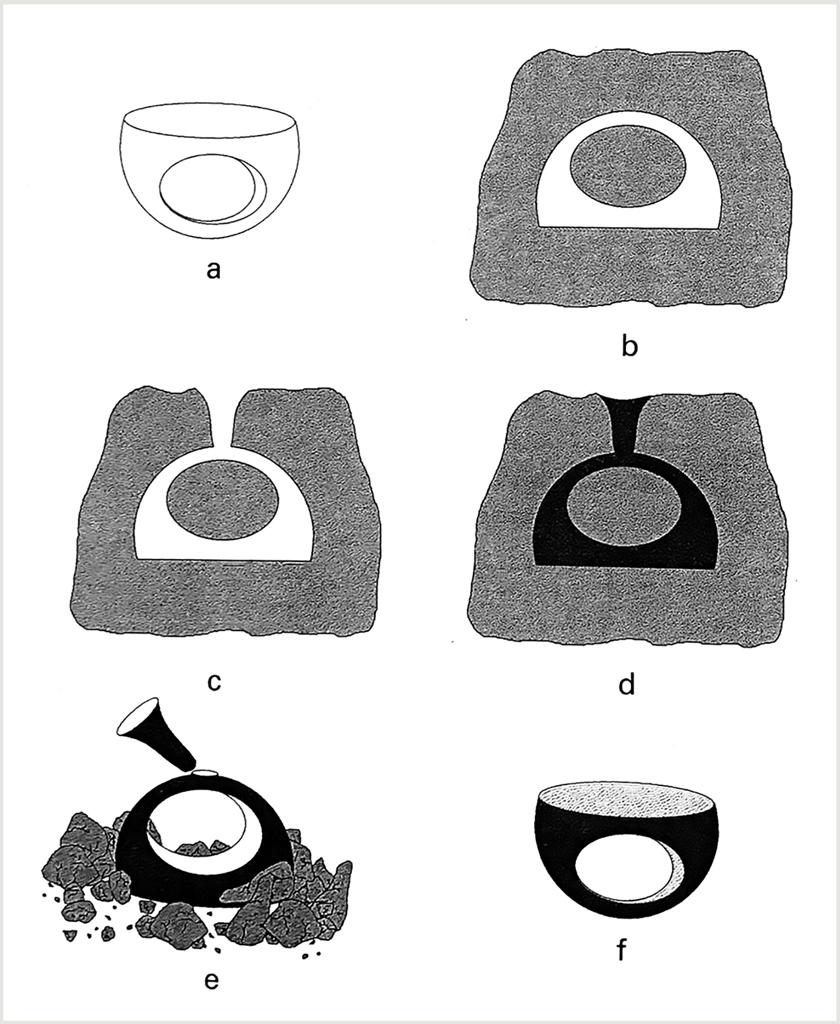The image depicts a detailed six-step diagram illustrating the transformation of a half-spherical shape with a cutout center, labeled from A to F against a gray background. The initial image, A, features a white, bowl-like drawing with a flat top and rounded bottom, notably having a large central hole rendering it non-functional as a bowl. Moving to B, this same shape is inverted and appears embedded in a piece of stone, presenting the negative space of the original form. In C, the upper section of the stone has been removed to expose the hollowed out top of the half-sphere. Image D fills all empty space with black, accentuating the original shape in contrast. E further advances the transformation by showing the stone entirely chipped away, leaving the isolated form that almost suggests a handle at the lower part. Finally, F reiterates the original half-spherical shape akin to A, but now depicted in black and slate gray, maintaining the defining features of a flat top, rounded bottom, and central hole.